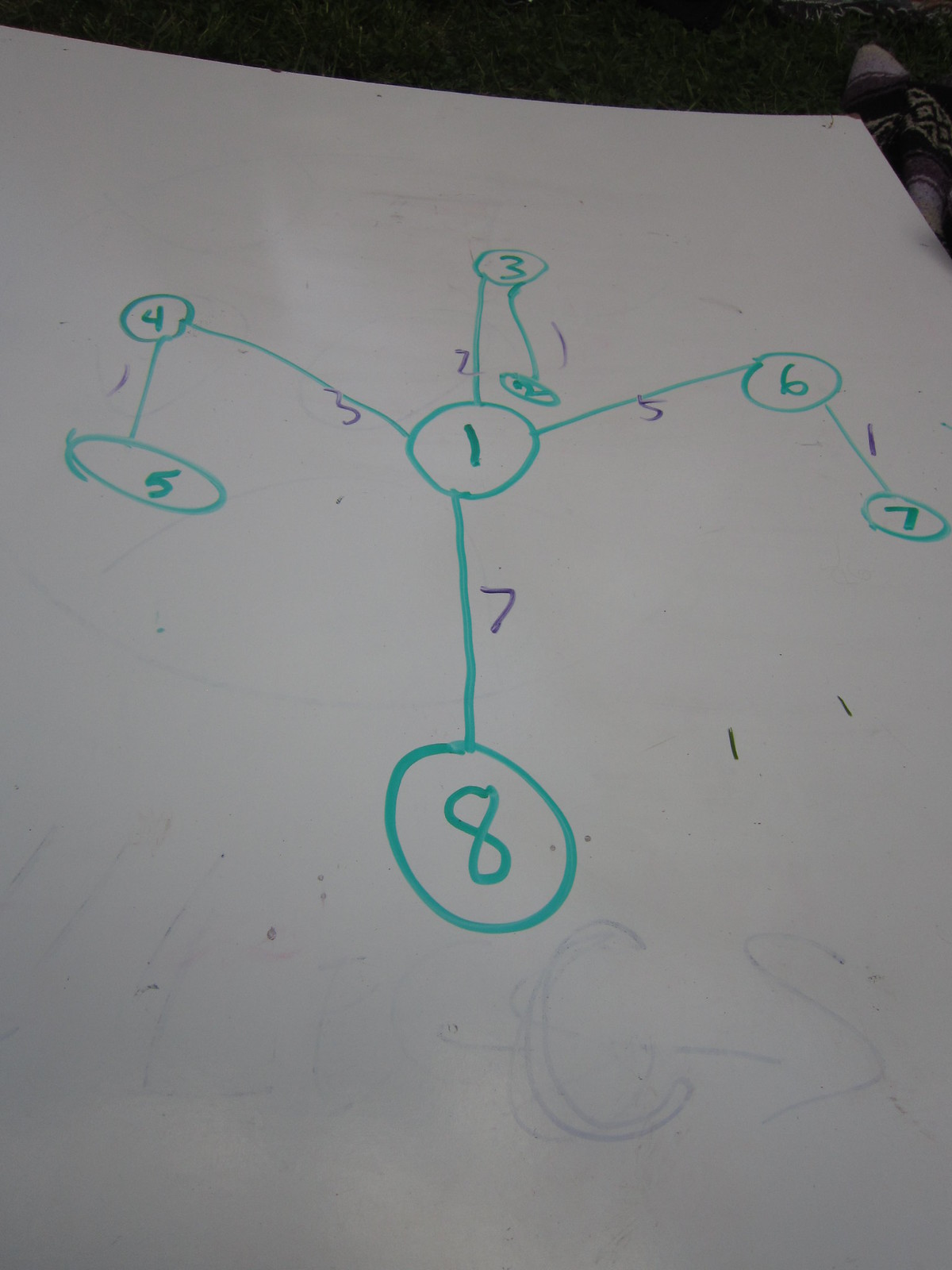The photograph showcases an illustration drawn on an expansive white sheet of paper, which contains some faint markings and gray shadowing. Towards the bottom of the sheet, there are faint, grayish letters "C" and "S." The central illustration, rendered primarily in green ink, consists of a series of interconnected circles and numbers. A circled green number "1" serves as the focal point at the center of the image.

Radiating from this central "1," a line extends to a circled "4" and continues to a circled "5" below it. Above the "1," a circled "3" is connected by a line, with a circled "2" directly beneath it. Below the central "1," a line leads down to a circled "8." Extending to the side from the "1," a circled "6" is connected, with a circled "7" situated below it.

The green lines and circles are interspersed with additional numbers in a purply-blue hue, alongside several other numbers, including 3, 5, 7, and what appears to be a 2, scattered around the drawing.